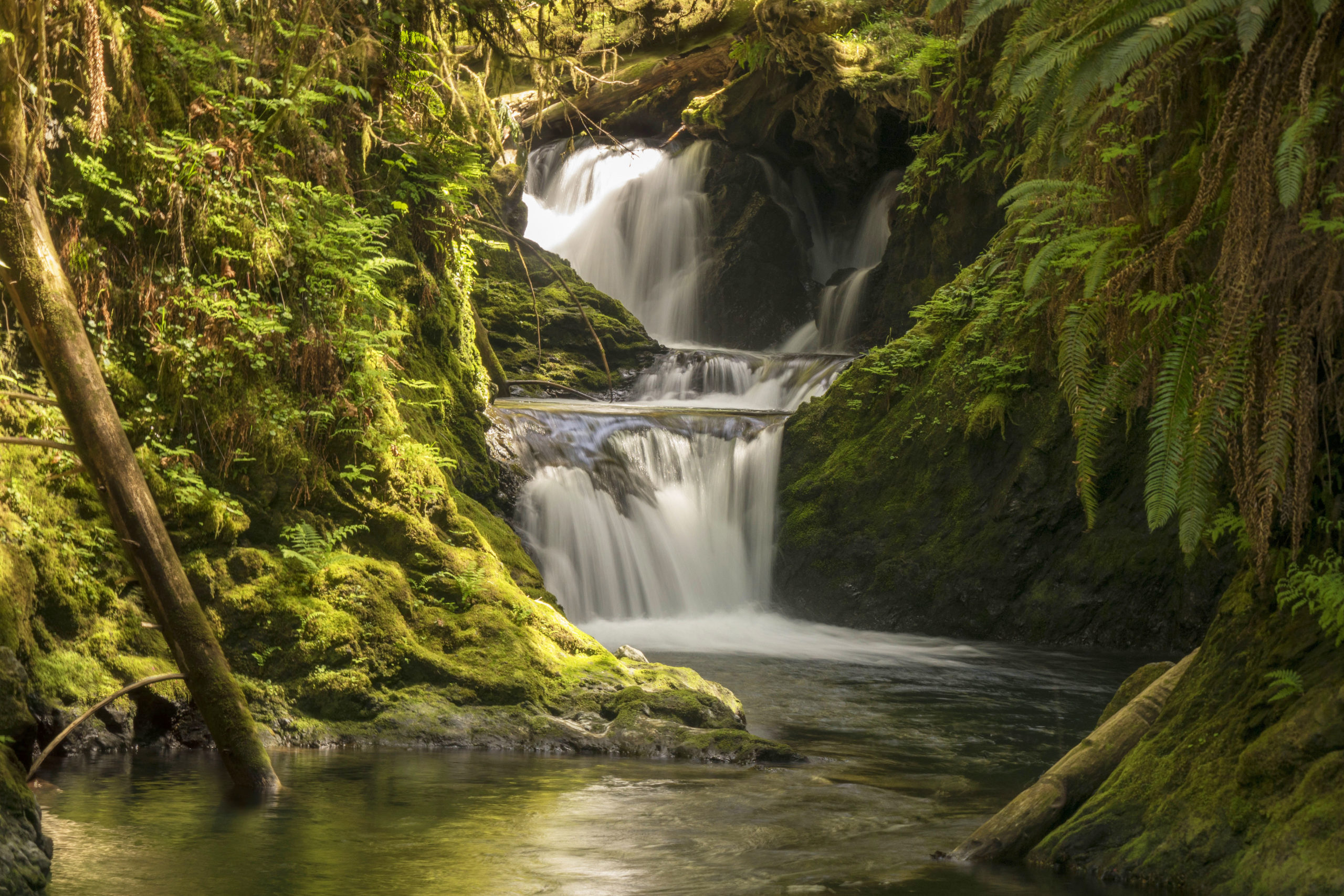This stunning landscape photograph captures a serene forest scene dominated by a cascading waterfall. The image, presented in a rectangular layout slightly longer than it is tall, features lush greenery with an abundance of green leaf trees, ferns, and moss-draped branches on both the right and left sides. In the center, the waterfall descends in tiers – first cascading into a small pool, fed by a second tributary, before plunging again into a larger pool at the bottom of the image. The water is crystal clear, revealing brownish hues from the rocks beneath its surface. The forest is dense with trees, including visible tree trunks and partial branches interspersed among the vibrant foliage, creating a verdant tapestry with occasional brown highlights from the tree bark. The overall scene presents a tranquil and untouched natural setting with no human presence, emphasizing the purity and beauty of nature.